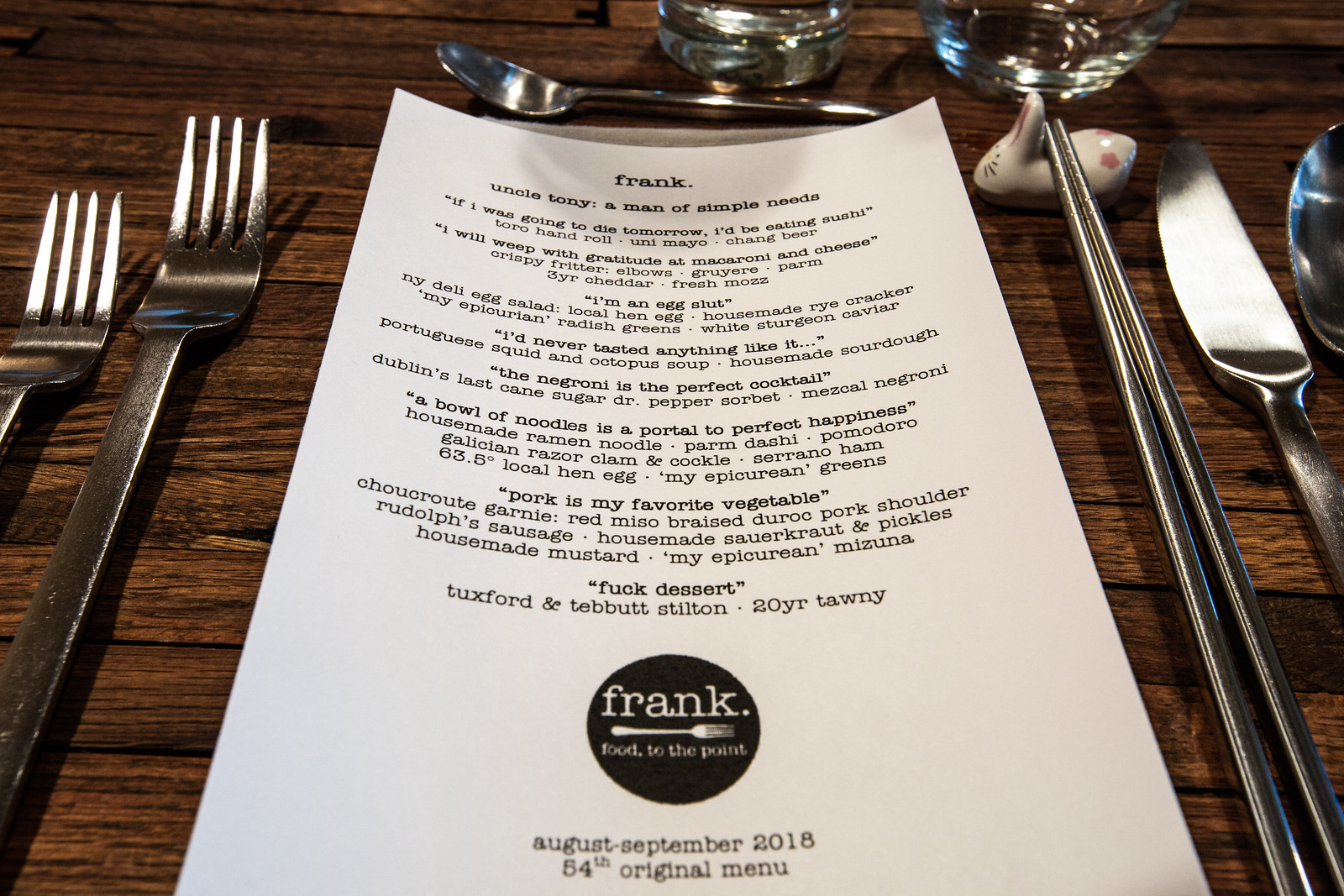In this captivating image, we see Uncle Tony—a man of simple needs—sitting at a well-set dining table. He is contemplating a diverse and luxurious menu filled with his favorite gourmet dishes, expressing gratitude for each delightful option. The menu includes an array of exquisite foods: sushi Toro hand rolls topped with uni mayo, paired with a Chang beer, and macaroni and cheese made with crispy fritters and three-year cheddar. Among the intriguing options is a dish called "Egg Slut," featuring an egg salad made with a local hen egg, house-made rye cracker, radish greens, and white sturgeon caviar.

Further down the menu, there's Portuguese squid and octopus soup served with homemade sourdough bread. The Negroni cocktail is praised for its perfection, made with Dublin's last cane sugar Dr. Pepper. A bowl of house-made ramen noodles with parm dashi pomodoro, Galician razor clams, cockles, serrano ham, and a local hen egg promises to be a portal to perfect happiness. Uncle Tony mentions that pork is his favorite vegetable and expresses an aversion to dessert with a humorous comment at the bottom of the menu.

The table is elegantly set with silverware on the left and right, ready for a feast that perfectly captures Uncle Tony’s love for fine food and simple pleasures.